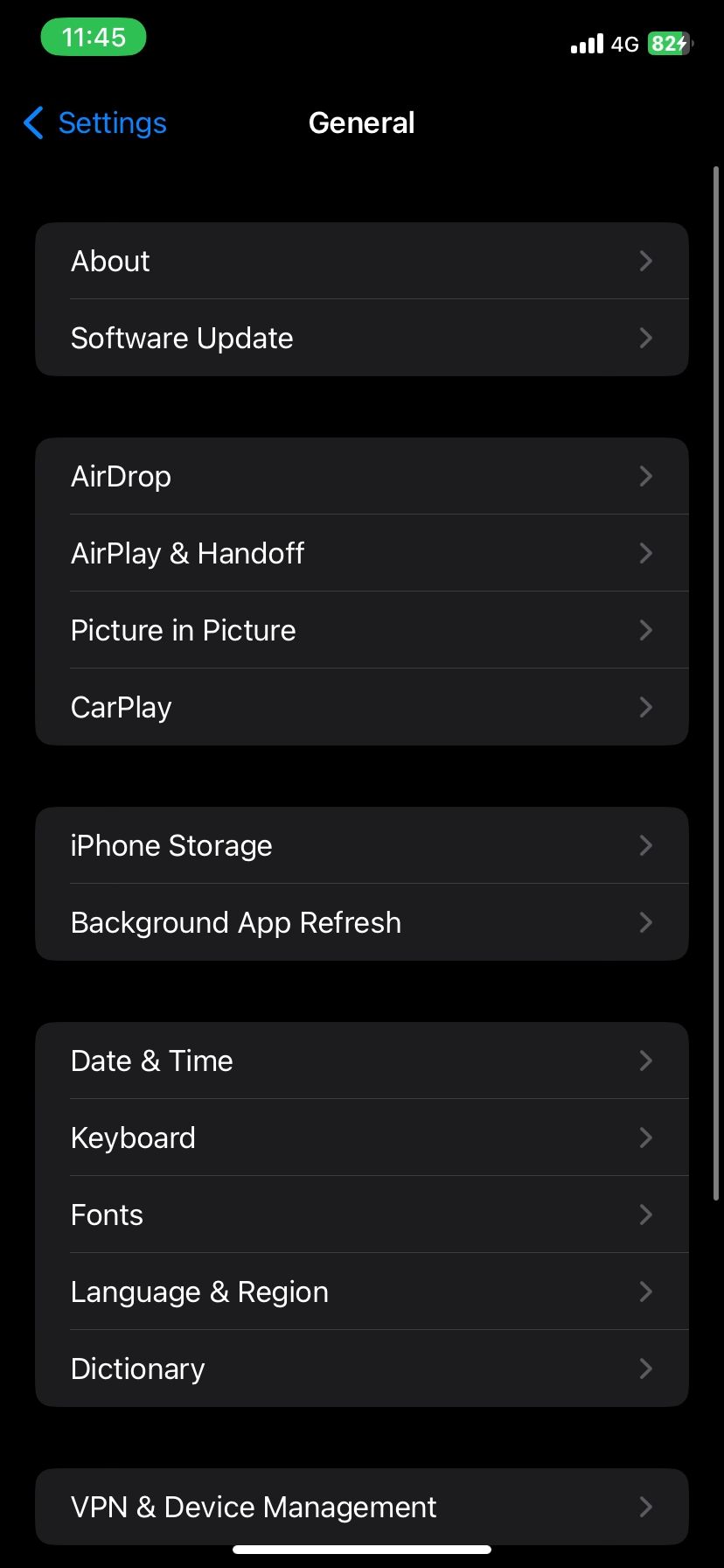This is a detailed caption for the provided image:

---

A dark mode screenshot of the General Settings menu in a recent version of iOS. The interface is set to English and the time displayed at the top of the screen is 11:45 AM. The status bar shows a strong 4G signal and the battery is currently charging at 82%. The settings options visible on the screen include: "About," "Software Update," "AirDrop," "AirPlay & Handoff," "Picture in Picture," "CarPlay," "iPhone Storage," "Background App Refresh," "Date & Time," "Keyboard," "Fonts," "Language & Region," "Dictionary," "VPN," and "Device Management." The upper left corner features a light blue circular background, highlighting the general settings of the iOS. This menu allows users to access further sub-pages for detailed configurations of their device.

---

This caption provides a comprehensive and clear description of the screenshot, making it easier for anyone to understand the contents and layout of the image.